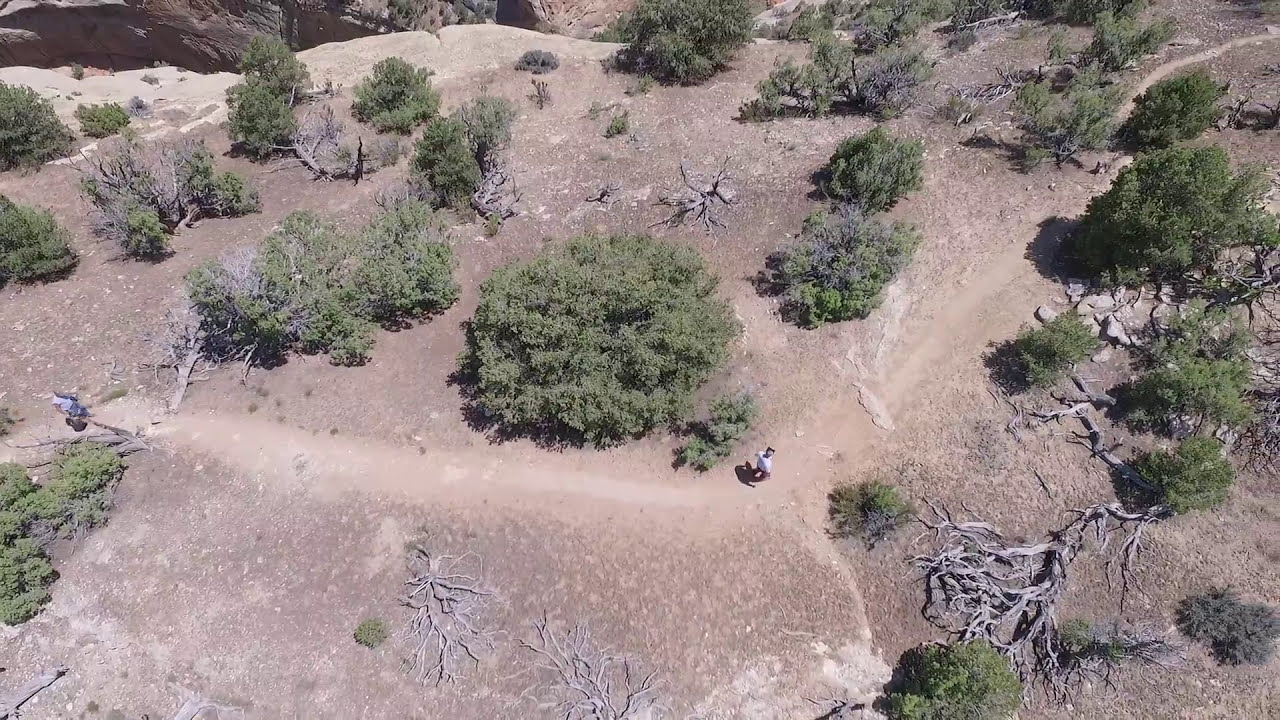This aerial photograph captures a rugged and arid landscape featuring a network of dirt hiking paths traversing the rocky, barren terrain. The ground is dotted with scrub brush and patches of greenish vegetation, interspersed with large bushes and trees with exposed roots and dead branches. Several individuals can be seen walking along the paths that cut through the light yellow, dusty hillsides. Amongst the trails, scattered rocks act as steps or obstacles, typical of hiking trails found in Southern California or the deserts of Utah or Arizona. The top of the image showcases some whitish-yellow rock formations that appear to drop off sharply, suggesting the edge of a cliff. On the left side of the image, there's a blue and white object, likely a person or a misplaced item. The overall scene conveys a dry, rugged environment with sparse vegetation, capturing the essence of an arid outdoor adventure.